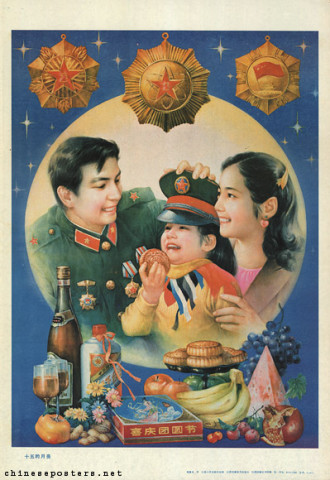The product poster, set against a white, featureless void to emphasize its contents, is displayed in a commercial style suited for online shops, catalogs, or websites. The rectangular poster has dimensions where the length is twice the height and features a light gray border around its edges. The bottom left corner is marked with black text reading "ChinesePosters.net." The majority of the text on the poster consists of blue Asian characters. The central image vividly portrays a smiling uniformed man, adorned with badges, placing his hat on a small child who is eating a piece of bread or doughnut. The child is warmly embraced from behind by a woman, who is also smiling. In front of them, a bountiful display of food can be seen, including doughnuts, bananas, cakes, grapes, and a bottle of wine or champagne. The background of the image within the poster is blue.